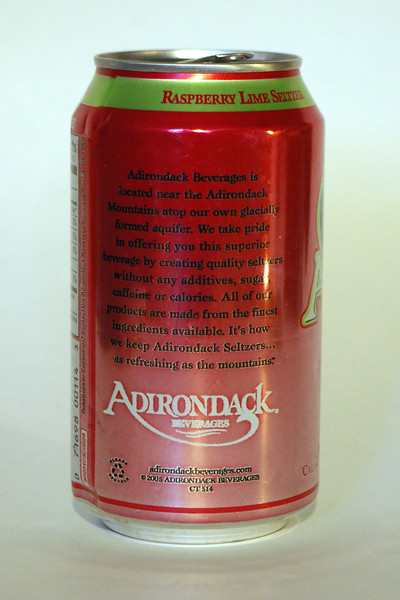The image depicts a vertically-shot, red Adirondack Raspberry Lime Seltzer can against a white background. The can features a lime green line around the top, near the lip of the lid, and a green banner at the very top with "Raspberry Lime Seltzer" printed in red letters. The visible side of the can includes the beverage's description in black, emphasizing its purity, stating that the beverage contains no additives, sugar, caffeine, or calories and is made from high-quality ingredients sourced from a glacially formed aquifer near the Adirondack Mountains. Near the bottom of the can, in white stylized font, the Adirondack Beverages logo is prominently displayed, with a recycling symbol to the left and additional company information, including their website address, centered below it. A hint of the nutritional facts label can be seen to the left, while a partial "A" peeks from the right, indicating the front side of the can.